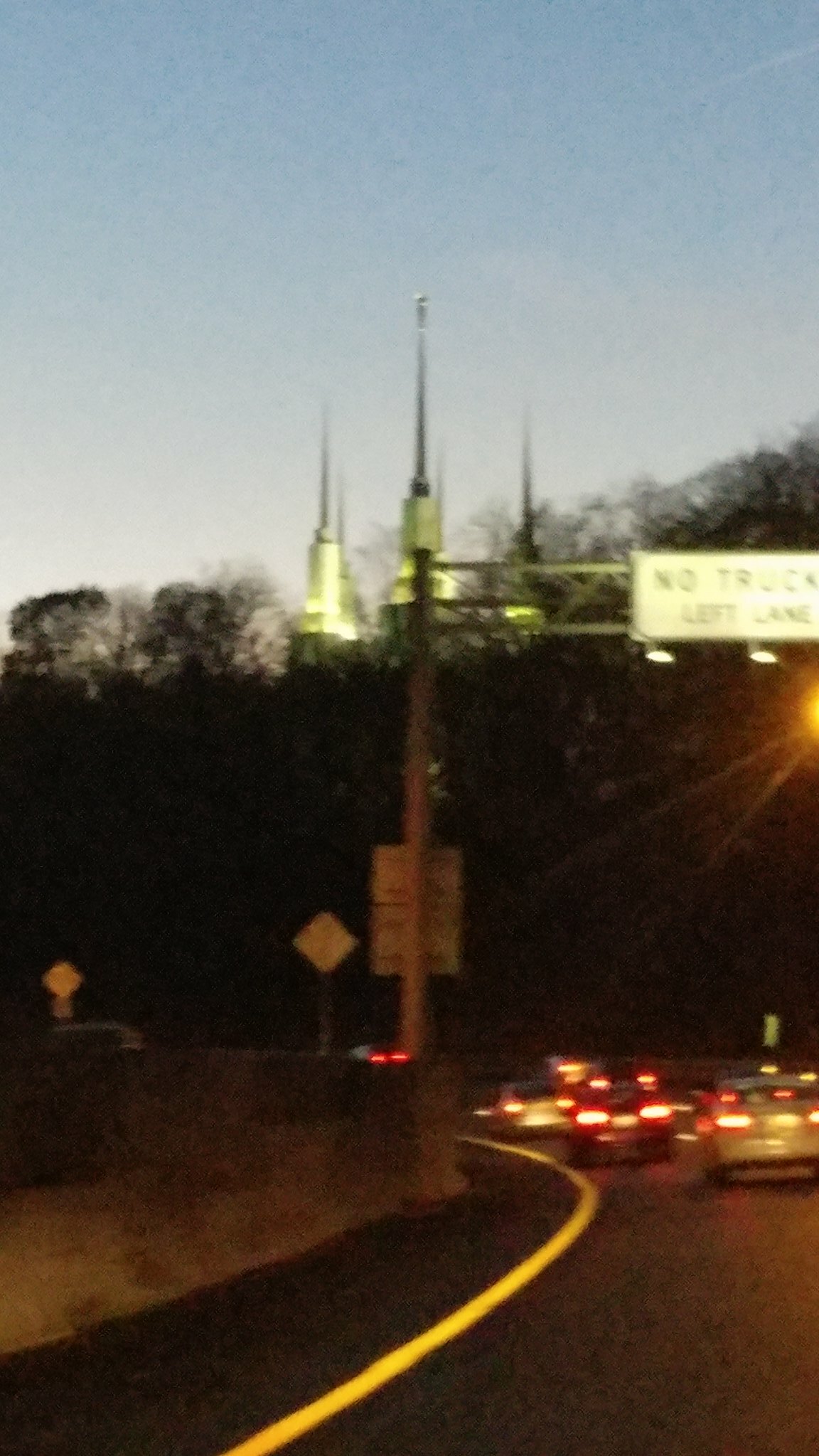The image is a vertical, rectangular photograph taken outdoors, capturing a scene likely during dawn or dusk. The top of the image shows a light blue sky that gradually fades into white near the horizon, speckled with a few white clouds. In the far distance, three tall spires or towers, colored in white and black, stand silhouetted against the sky, though their exact nature is unclear. The foreground features a line of dark trees, possibly due to the shadowing from the low sun, adding to the twilight ambiance of the scene.

The photo is slightly out of focus, but it distinctly shows a black asphalt highway running across the bottom and right side of the image. The yellow lines on the road curve from the bottom left and then back toward the left. A gray road median and some patches of what appears to be grayish-yellow grass or a grassy area can be seen on the left. Positioned towards the middle right side, a vertical, gray traffic sign with horizontal bars and a rectangular white sign attached to it bears the message "No Truck Left Lane" in black letters.

There are approximately ten cars visible on the highway, most of them showing red taillights which suggest they are slowing down. Some cars appear dark-colored while others are gray. The scene is lit by ambient light, reflecting the transitional time of day, enhancing the serene yet slightly blurred view.